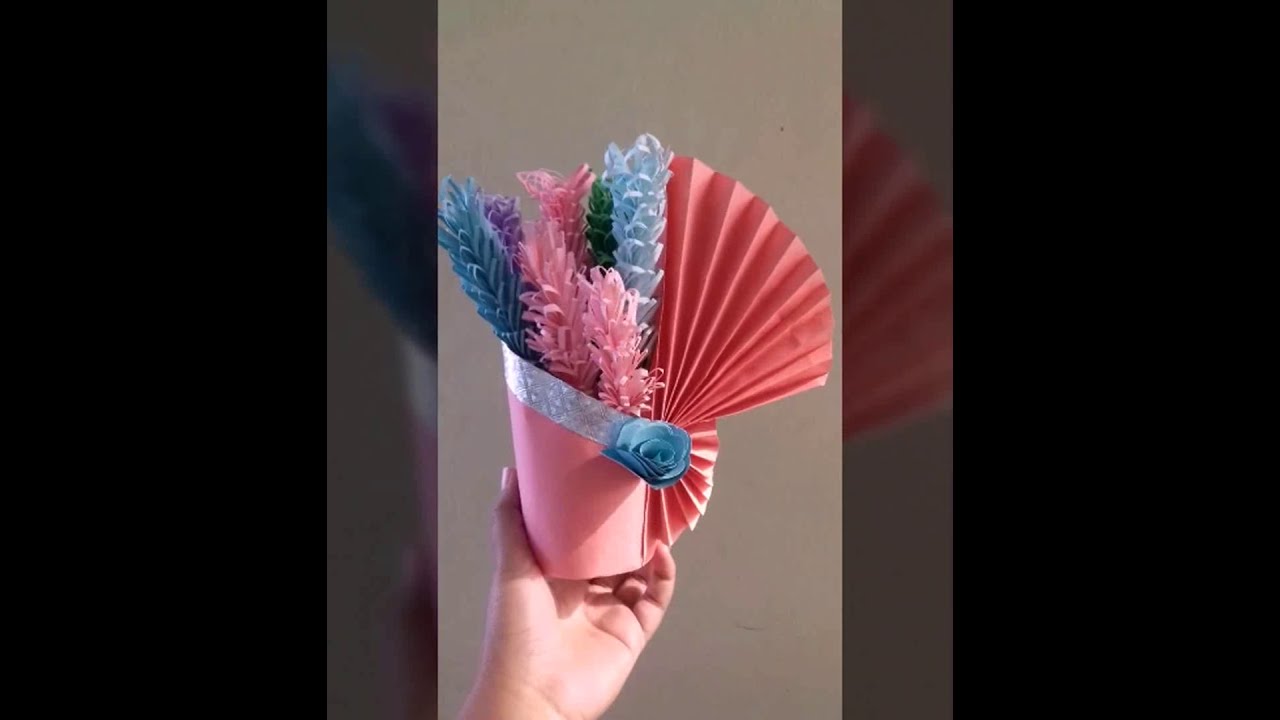In the image, a person is holding a hand-crafted origami vase adorned with various colored paper flowers. The vase, primarily pink, features a pleated or fan-like detail on one side, folded meticulously to create an elegant pattern. Around the top part of the vase, a silver strip ties it together, with a blue rose-like paper flower accentuating one side. Nestled inside the vase are seven paper flowers: three pink, two light blue, one green, and one purple, resembling delicate flower buds with no visible stems. The person's hand, emerging from the lower left corner, supports the vase, illuminated by a light source from the upper right, highlighting the palm and fingers. The background is dull and desaturated, encased in a thin, blurred border that blends into thicker black borders on the left and right sides.